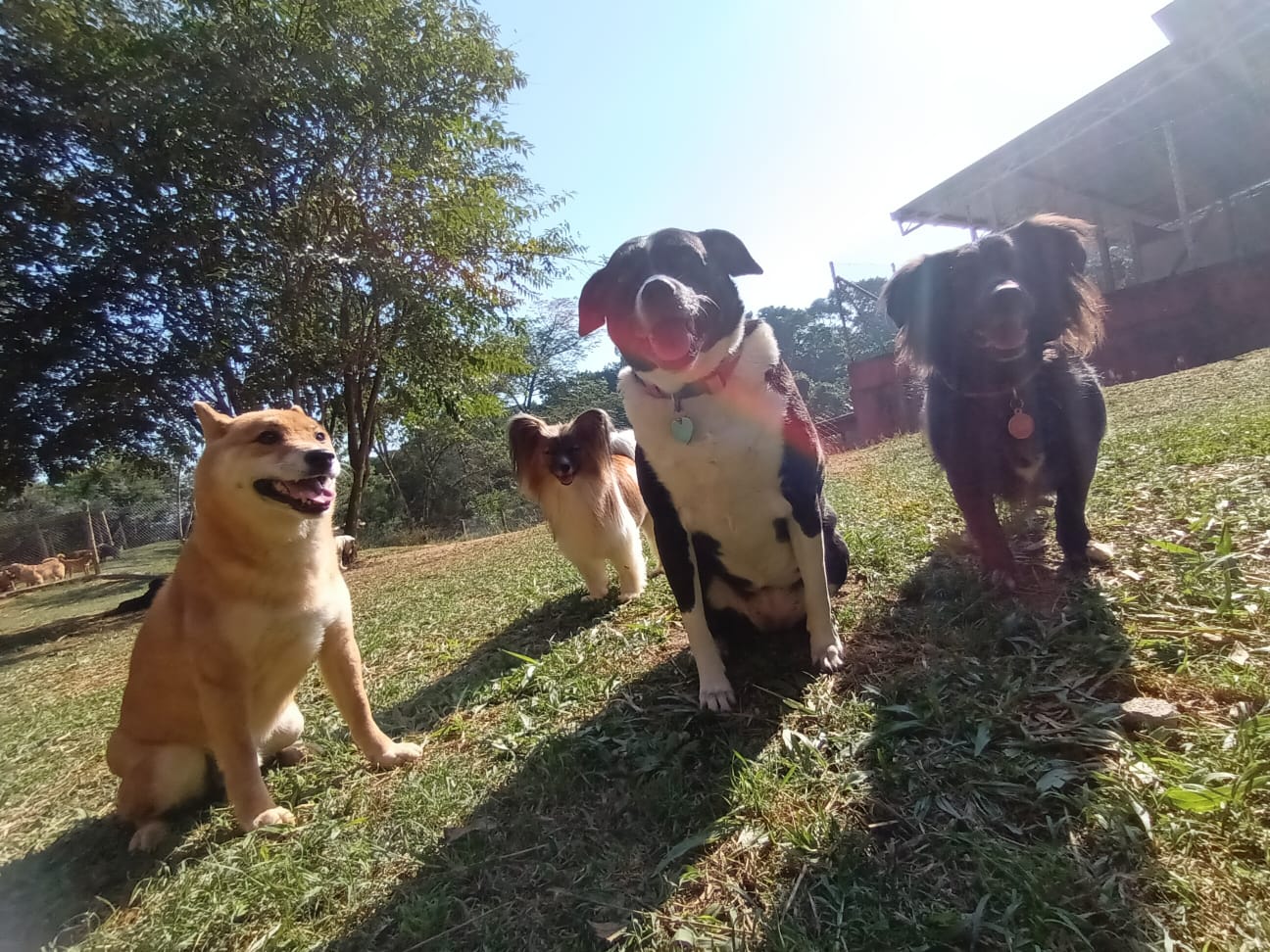In this captivating photograph taken from a ground-level, dog's-eye view, four excited dogs are captured in a yard, exuding post-play energy as they pant with contentment. From left to right, the first dog is a small, golden and white Shiba Inu, sitting and gazing off-camera, its fur illuminated by the sunlight. Behind this Shiba Inu is another smaller, furrier dog, distinguished by its black and white coat and spotted markings. Moving further right, the third dog, the largest and positioned closest to the camera, shares similar black and white coloring with a white nose and black face, and wears a collar adorned with a heart-shaped pendant. Concluding the lineup on the far right is a darker all-black dog, standing with a collar and a circular-shaped pendant, its face obscured by the sunlight streaming from behind. The backdrop of the photo includes a yard with patches of green and brown grass, a tall tree dominating half of the background, other trees scattered in the distance, and a white, wall-less garage structure. The first and third dogs sit while the second and fourth dogs stand, creating an engaging dynamic that captures the essence of their varied personalities.